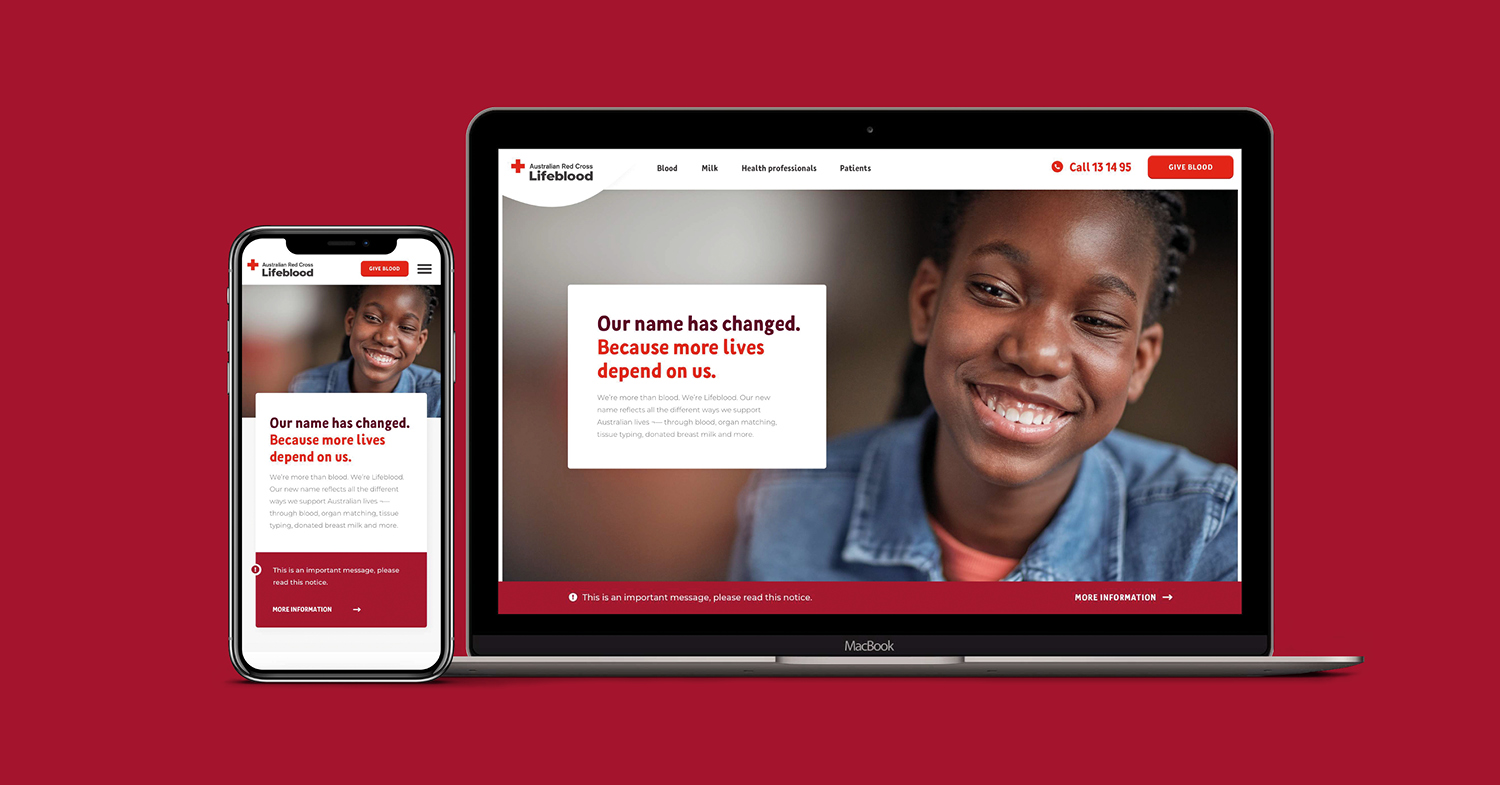This image features a web page displayed on both a smartphone and a laptop screen, showcasing the Lifeblood website. The layout of the website prominently includes what appears to be the Red Cross logo positioned on the left. To its right are four navigation tabs, the text of which is not legible. Further right is a contact phone number, accompanied by an opaque orange button with indistinguishable text. 

The web page features a prominent pop-up box reading, "Our name has changed because more lives depend on us," overlaying an image of a smiling young African girl. She is wearing a denim jacket over an orange blouse and her hair is styled in braids. The laptop displaying this web page is a MacBook with a black screen border and a grayish cover. The smartphone has a chrome finish border, mirroring the exact same web page image seen on the laptop.

At the bottom of the web page is a burgundy border, adding a final touch to the website's design. The website name, Lifeblood, is presented as one word, emphasizing its branding.